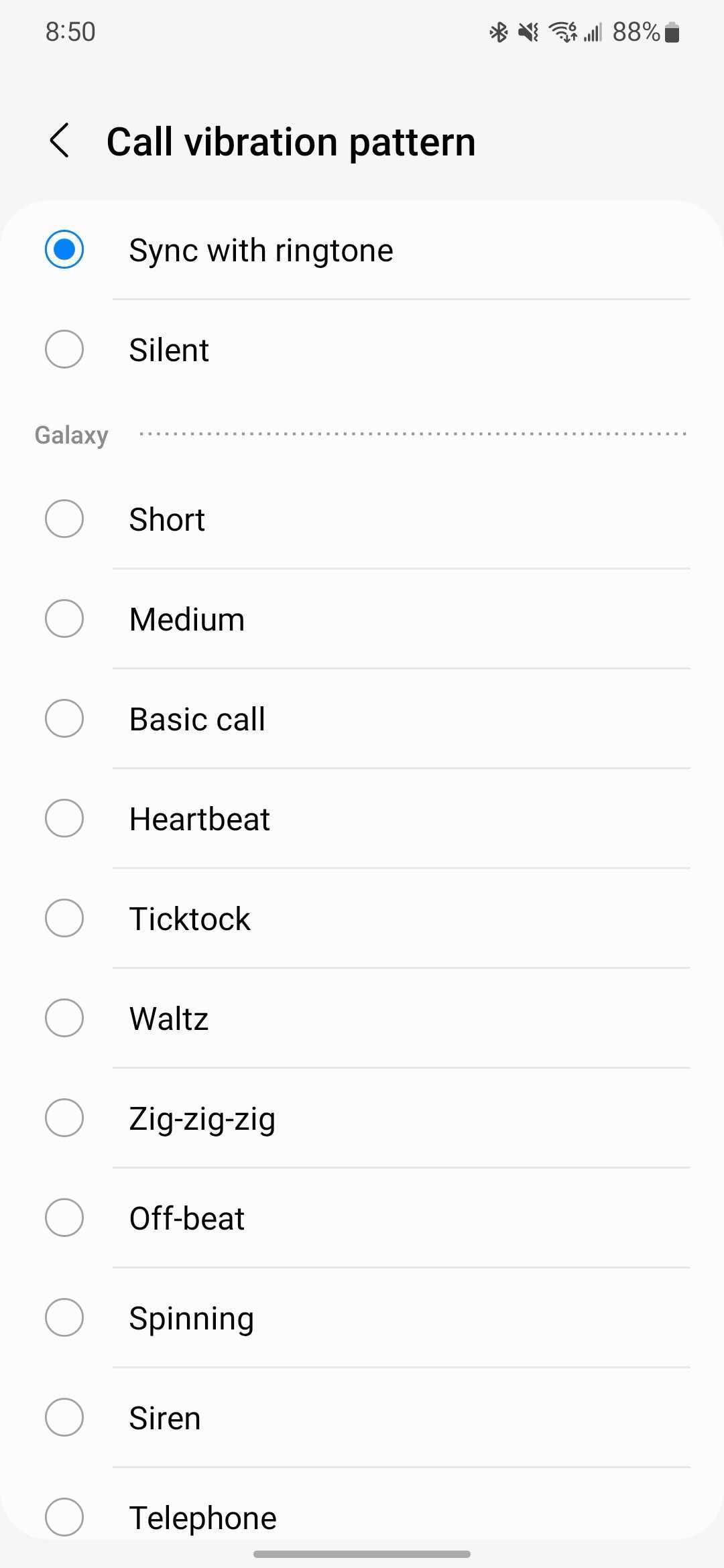This image, captured on a smartphone screen, displays the "Call Vibration Pattern" settings page. At the top of the screen, the status bar indicates the phone's battery is 88% charged, shows a good network connection, and the current time is 8:50. 

On the page, there are two primary options under the heading "Call Vibration Pattern": "Sync with Ringtone," which is highlighted in blue, indicating it is currently selected, and "Silent," which is unselected. Below these, there are multiple vibration pattern options listed vertically, including "Galaxy," "Short," "Medium," "Basic Call," "Heartbeat," "Tick Tock," "Waltz," "Zig Zig Zig," "Offbeat," "Spinning," "Siren," and "Telephone." Each option has an empty circular selection marker next to it except for "Sync with Ringtone," which is filled in blue to show it is active.

The entire list appears on a light gray background, with the user able to customize their phone’s vibration pattern by tapping on any of the empty circles to select their preferred option. This interface allows the user to set different vibration patterns for phone calls and texts, providing tailored notifications for their device.